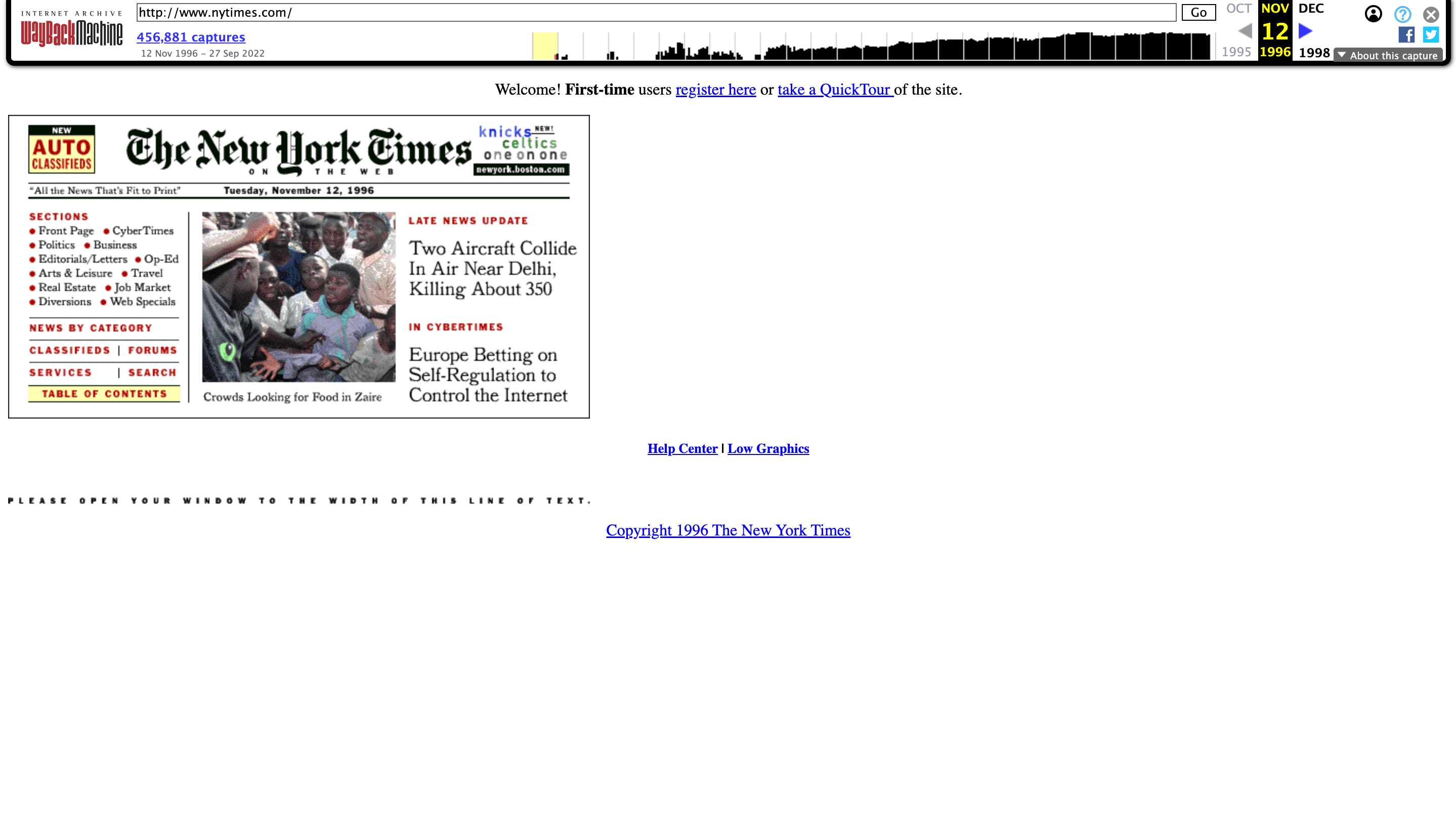A detailed description of this image could be:

"Displayed in the image is an archived version of the New York Times webpage, capturing its appearance on Tuesday, November 12th, 1996. This vintage snapshot features a minimalist design characteristic of early internet webpages. Dominating the top of the page is a small square logo that mirrors the iconic masthead seen in the print version of the New York Times, utilizing the same distinctive font and layout.

Beneath the header, the majority of the webpage appears blank, showcasing the simple and uncluttered user interface of the time. Key interactive elements are clustered at the top and bottom areas, including links for the Help Center, an option for low graphics, copyright information, and directives to register or take a tour of the website.

This historic capture highlights not only the evolving design trends in digital media but also offers a nostalgic glimpse into the early days of digital news consumption, emphasizing major headlines and providing users with essential navigational tools within a sparse and streamlined online environment."